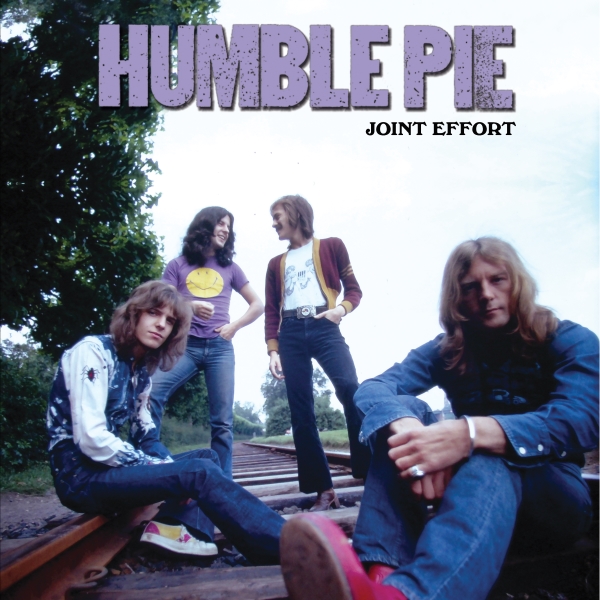This album cover from the late 1960s English rock band Humble Pie features a square, five-inch-by-five-inch photograph taken outdoors on train tracks. At the top of the image, in large purple letters, the band’s name “Humble Pie” is prominently displayed, with the album title “Joint Effort” just below in smaller black letters. The scene is set against a mostly white sky, with the upper left corner dominated by a tree.

In the lower right-hand corner, closest to the camera, a man of Caucasian descent with long blonde hair is seated on the railroad tracks. He wears a long-sleeve blue denim shirt, matching blue denim pants, and red boots. To his left, seated on the opposite side of the tracks, another man of Caucasian descent with long brown hair appears slightly younger. He sports blue jeans and a long-sleeve blue and white shirt, which features an image of a bug on the sleeve.

In the background, standing on the tracks are two men, both of Caucasian descent. The man on the right wears blue jeans and a vibrant red and yellow sweater over a white t-shirt, and has shorter dark brown hair. To his left stands another man with long dark brown hair, wearing blue jeans and a purple shirt adorned with a large yellow emoji on the front. They are facing each other, talking and smiling.